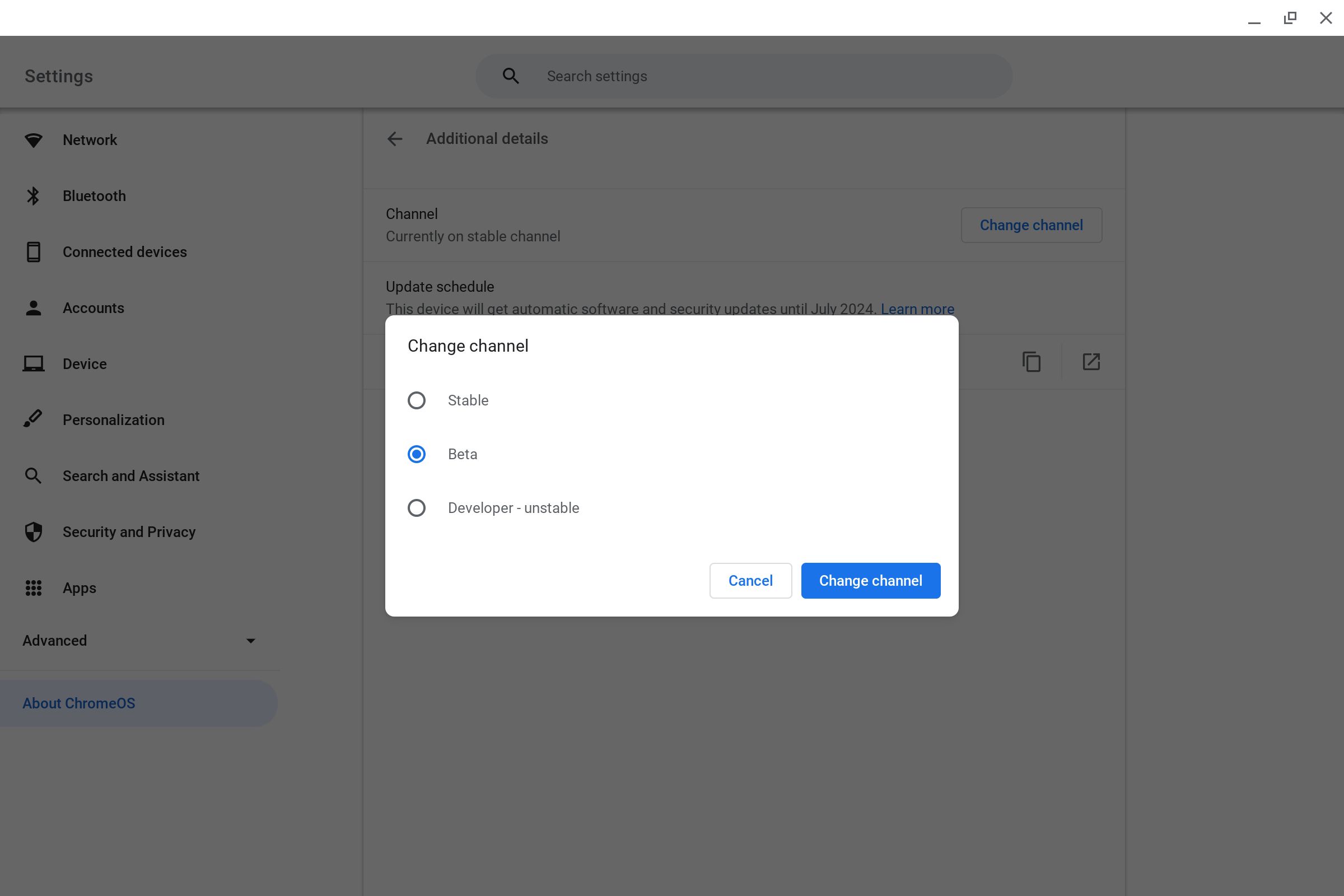This image displays the settings interface of the Chrome OS, highlighting the “Change Channel” feature. The central focus of the image is a white pop-up window, which partially grays out the main settings menu in the background. This pop-up window offers three radio button options arranged vertically: "Beta," "Developer (unstable)," and an unspecified third option. The "Beta" option is selected, indicated by a blue circle. At the bottom right of the pop-up, there are two buttons: "Cancel" (white font with blue background) and "Change Channel" (blue font with white background, highlighted for selection).

In the upper left corner sits a "Settings" tab, and at the top center, there's a back arrow with the word "Channel" below it, indicating the current view. Just under this, a line of text reads "Currently on the unstable channel," with a blue text button labeled "Change Channel" beside it.

On the left-hand sidebar, a vertical column of icons and labels provides navigation options, including "Network," "Bluetooth," "Connected devices," "Accounts," "Device," "Personalization," "Search and Assistant," "Security and Privacy," "Apps," and an "Advanced" section. Near the bottom of this sidebar, the "About Chrome OS" button is highlighted with blue font, suggesting it might be the current selection.

Above the sidebar is a search bar labeled "Search settings," enabling users to quickly find specific settings within Chrome OS. The detailed layout and color coding provide a clear and intuitive user experience for managing system preferences and updates on the Chrome operating system.